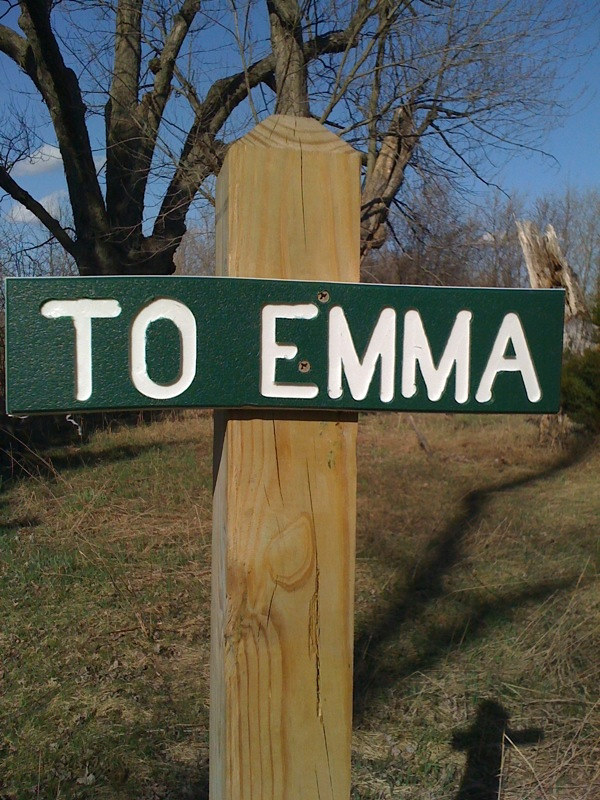A close-up image showcases a light brown wooden signpost firmly planted into the ground. The post, displaying visible wood grains, supports a green rectangular sign with white bold text that reads "to Emma," fastened with two screws. The green metal sign's shadow, cast to the bottom right, forms a cross-like shape on the burnt grass below. The background reveals a large, barren tree with intricate branches and twigs devoid of leaves, set against a blue sky dotted with a few white clouds in the bottom left corner. The ground features patches of burnt and green grass, further emphasizing the autumnal setting.